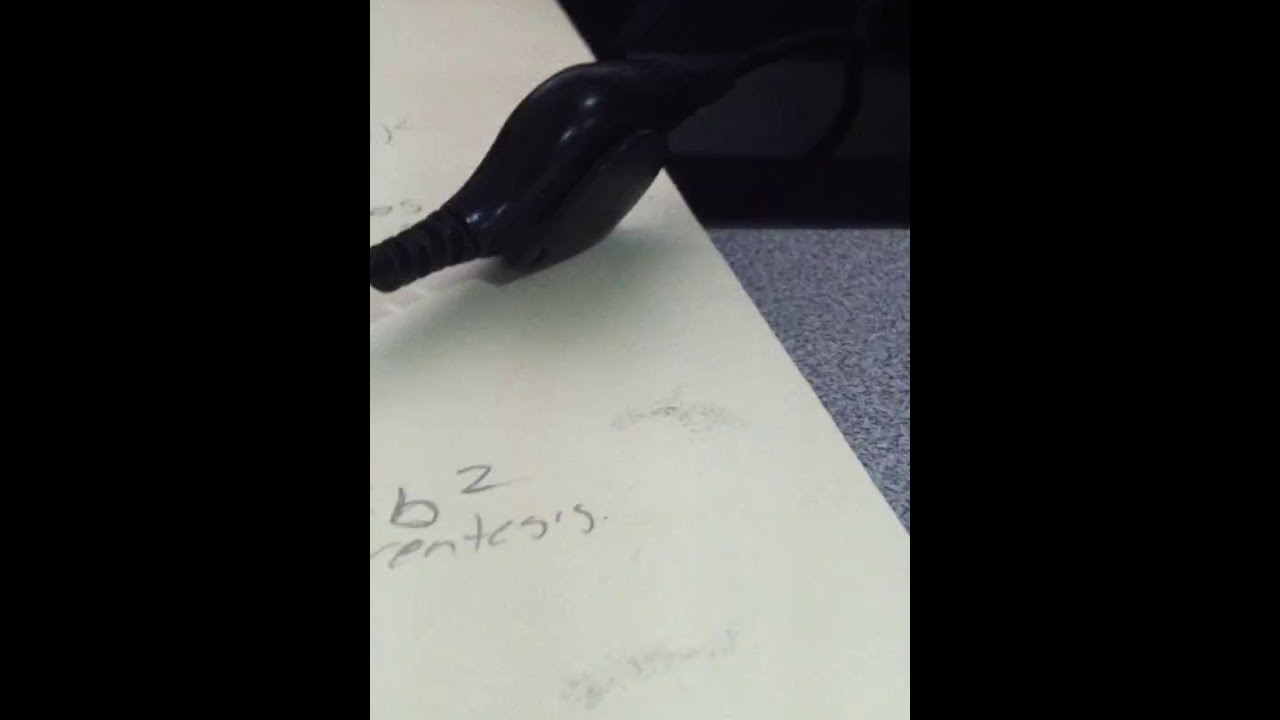The photograph showcases a close-up view of a somewhat cluttered tabletop scene. The backdrop appears to be a black and white or gray and white dotted textured table surface, possibly a granite or office tabletop. Dominantly, there is a piece of paper with a yellowish tint, scribbled on with 'B2ENTESIS' or a similar nonsensical word created in pencil, surrounded by numerous graphite smudges. The paper extends off the table edge, partially overshadowing the surface. Situated on the paper is a prominent black porcelain or glass figure resembling a bird with a round body, small feet, and a squared tail, although the head is indiscernible against the dark background. Accompanying this bird-like figure is a plastic control module, presumably a volume or mute selector for a set of headphones, marked by its rounded center and black cord extending in both directions. This detailed composition captures a moment of ordinary disarray, intertwining everyday objects into an enigmatic still life.